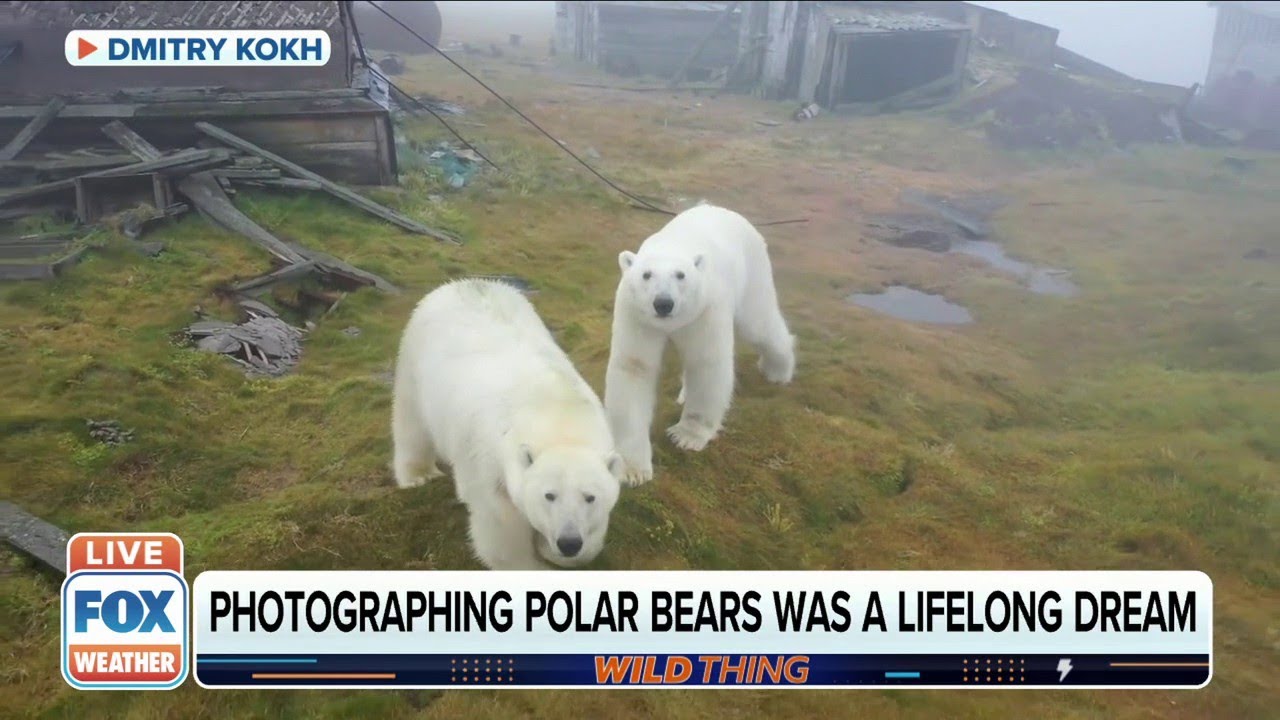This screenshot appears to be from a news channel video, showcasing a photograph in the background. The photograph captures an outdoor area with green and some brown grassy patches, featuring two white polar bears walking on a slightly hilly terrain dotted with puddles and rocks. The larger bear stands slightly in front of the smaller, both characterized by their black eyes, noses, and pointy ears. The surrounding environment includes several broken wooden houses, possibly due to a storm, and suggests a foggy day. In the top left corner of the screenshot, a white rectangle displays the name "Dmitry Kokh" in blue letters. The bottom center of the screenshot features centered all-caps black text reading "PHOTOGRAPHING POLAR BEARS WAS A LIFELONG DREAM," followed by all-caps red text "WILD THING." On the left side of the screen, there is a logo for "Fox Weather Live."